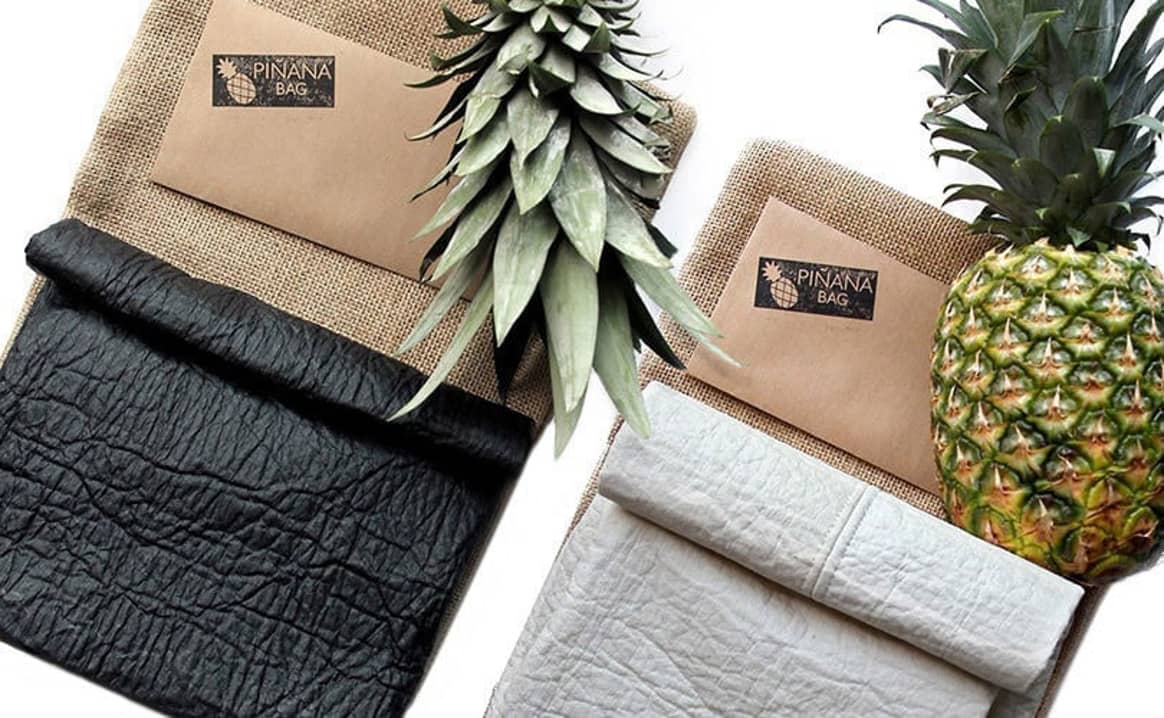This image features two Piñana bags displayed on a white background, positioned at an angle. Each bag has a beige flap and a crinkled body, with the left bag being black and the right bag being white. Both bags appear to be open, revealing tan cloth. Each bag is stamped with "PINANA BAG" in white capital letters next to a pineapple icon. The left bag showcases the upside-down leaves of a pineapple, while the right bag displays an entire green, not fully ripe pineapple with its leaves upright. These distinctive pineapple motifs emphasize the unique design of the Piñana bags.